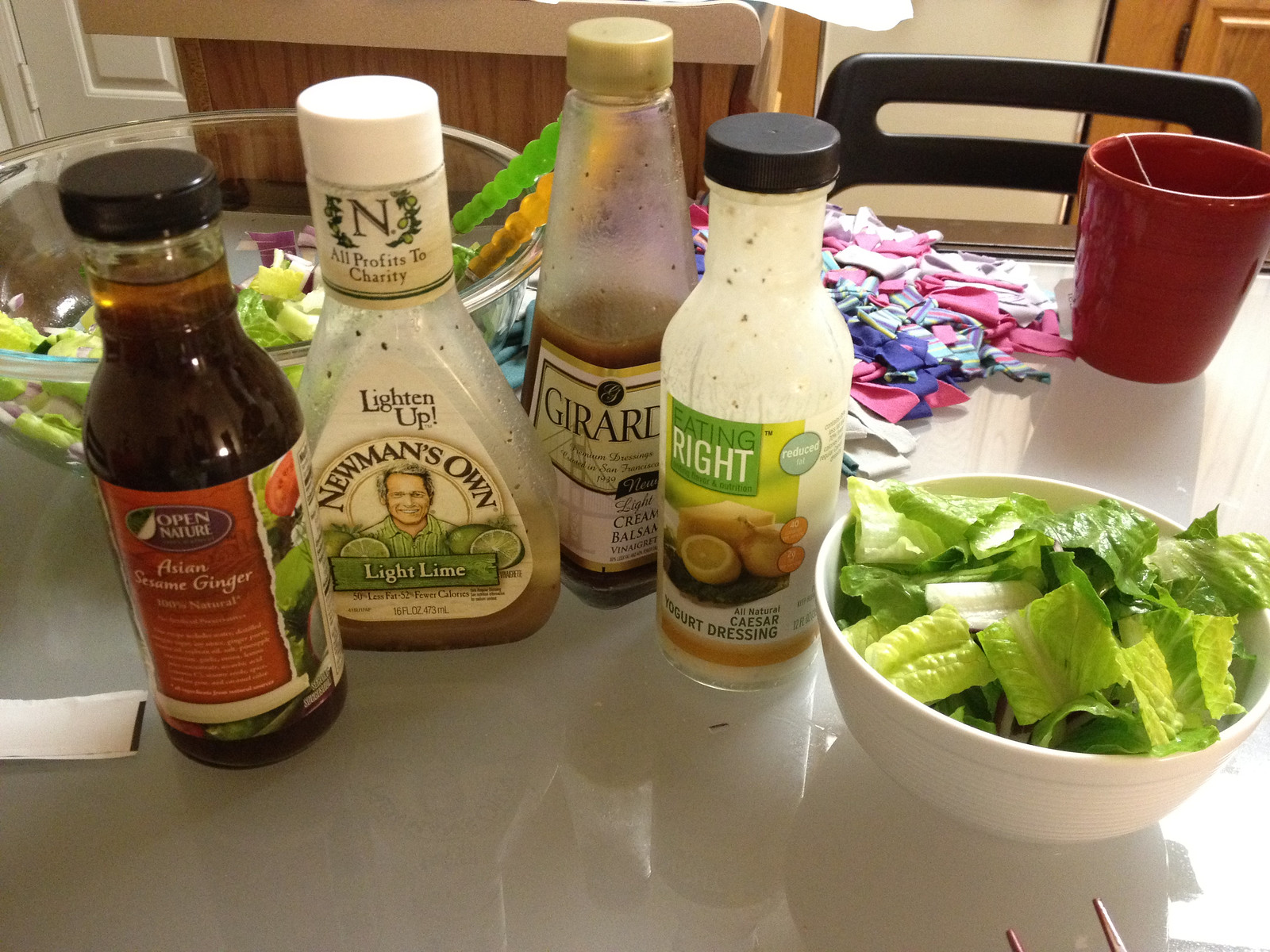In this photo taken from an overhead angle, we see a white, glossy kitchen table. On the top left corner of the table, a large clear glass bowl is filled with a fresh salad, accompanied by green and orange serving spoons. In front of this large salad bowl are four distinct jars of salad dressings neatly arranged: Newman's Own Light Lime with a white cap, which is about one-third full; a fully filled bottle of Asian Sesame Ginger dressing with a black cap; a Creamy Balsamic Vinegar dressing, half-filled and partially obscured behind the others; and a Caesar Yogurt Dressing. To the right of these dressings is a smaller white bowl, also filled with salad, prepared for an individual serving. On the top right part of the table, there is a red teacup with a teabag string hanging out. The setup is simple yet inviting, perfect for a healthy meal.